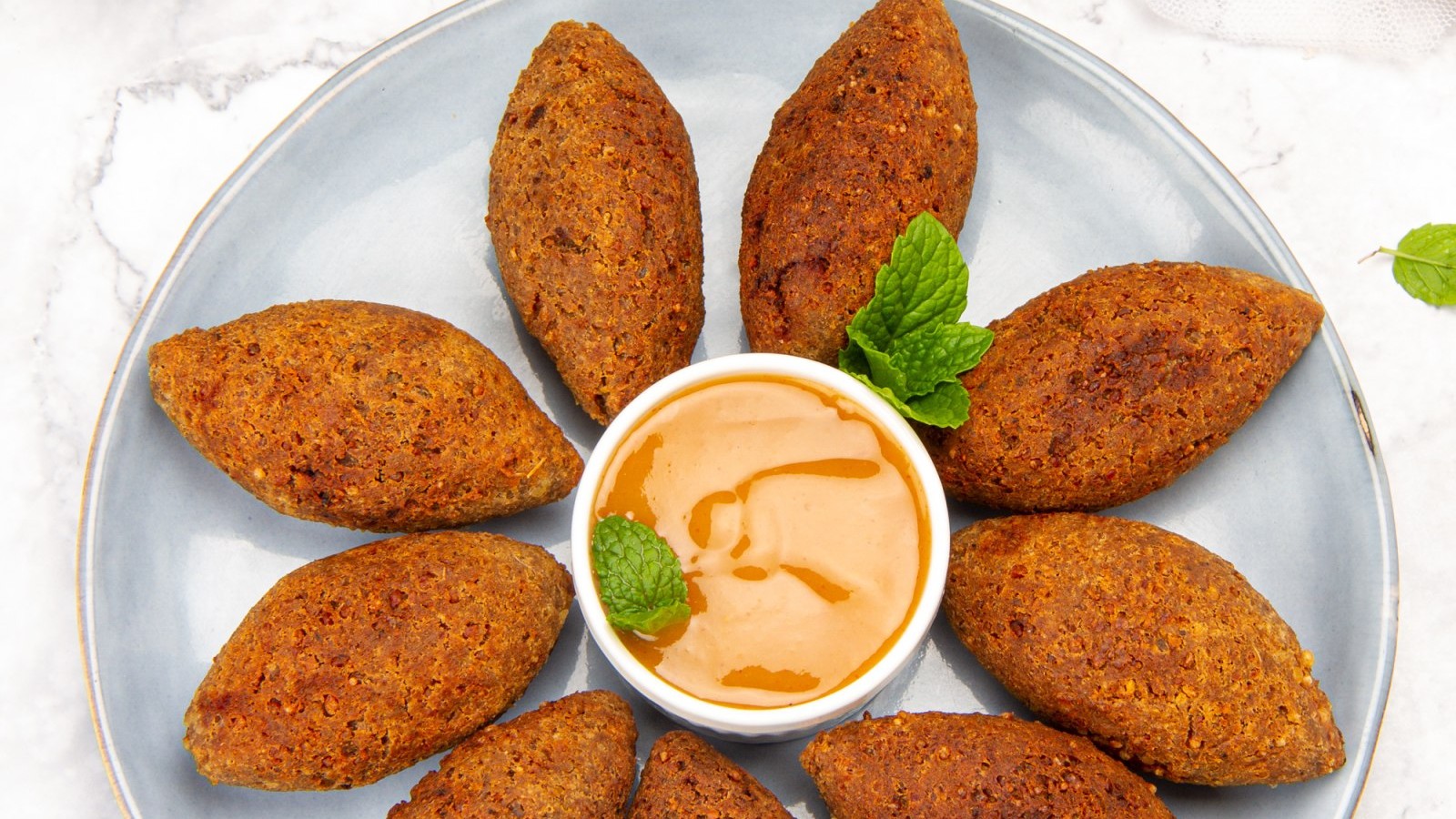In the image, a white plate with a silver edge is placed on a white marble countertop, garnished with small green leaves. The centerpiece is a small, round white bowl filled with a thick, orange sauce, topped with a green leaf. Arranged around the bowl are nine pieces of oval-shaped, breaded or fried food, resembling small footballs. The food items are evenly spaced in a circular pattern, creating a petal-like formation that mimics a flower. Additional green leaves are placed on some of the food pieces, with a stray leaf visible in the upper right corner of the counter. The meticulous arrangement and vibrant colors offer an aesthetically pleasing presentation.